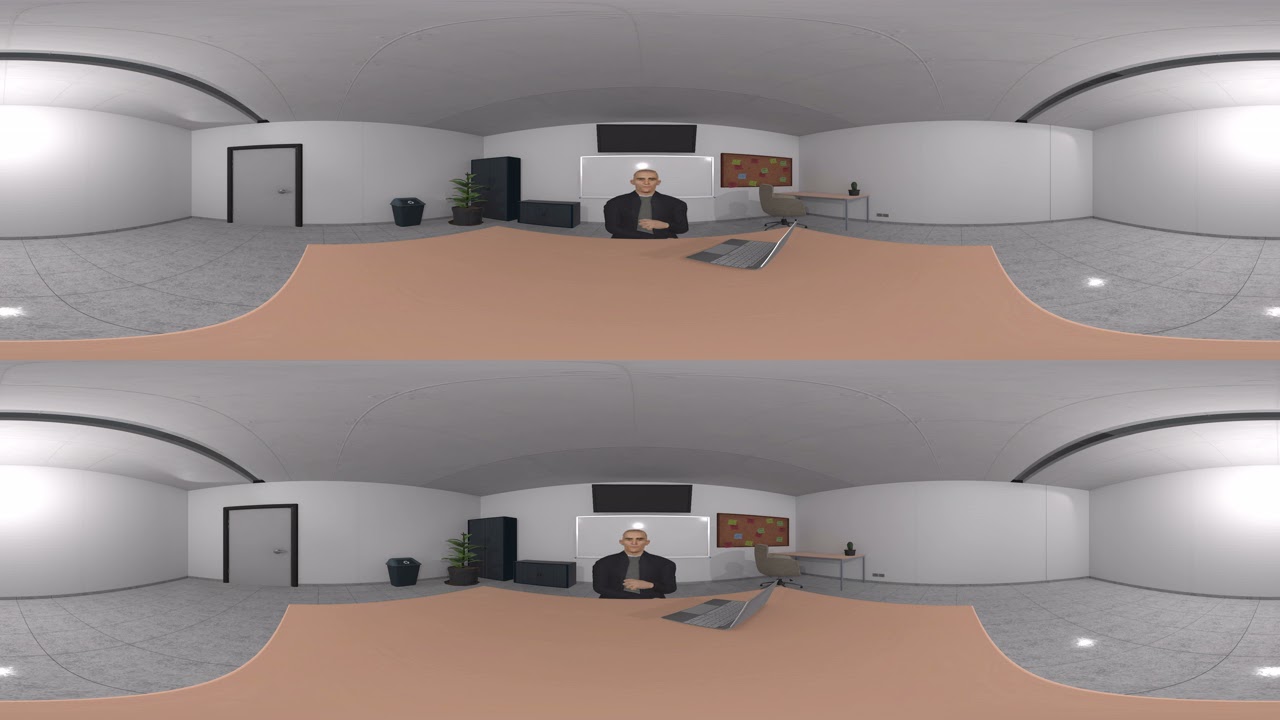The image features a well-lit, modern office room with white and light gray walls and a gray concrete floor. At the center of the scene is a large, wooden table with a laptop on top, and a bald man in a black suit jacket with a gray undershirt seated across from the table. The room displays a blend of minimalist and functional design elements. 

Behind the man, to his right, there is a whiteboard flanked by a bulletin board covered with red, green, and blue stickers. A flat-screen TV is positioned above the whiteboard. To the left of the whiteboard, a black indoor house plant in a black vase stands next to a black cupboard and a waste paper basket. In the left corner of the room, there's a smaller desk on adjustable wheels with an object placed on it.

The image is presented twice, one stacked atop the other, enhancing the panoramic perspective that shows both the curved walls converging at a seam and portions of the ceiling adorned with black rings following the wall curves. The room also features strategic lighting, with lights mounted on the walls and additional smaller lights on the floor in the far left and right corners of the image.